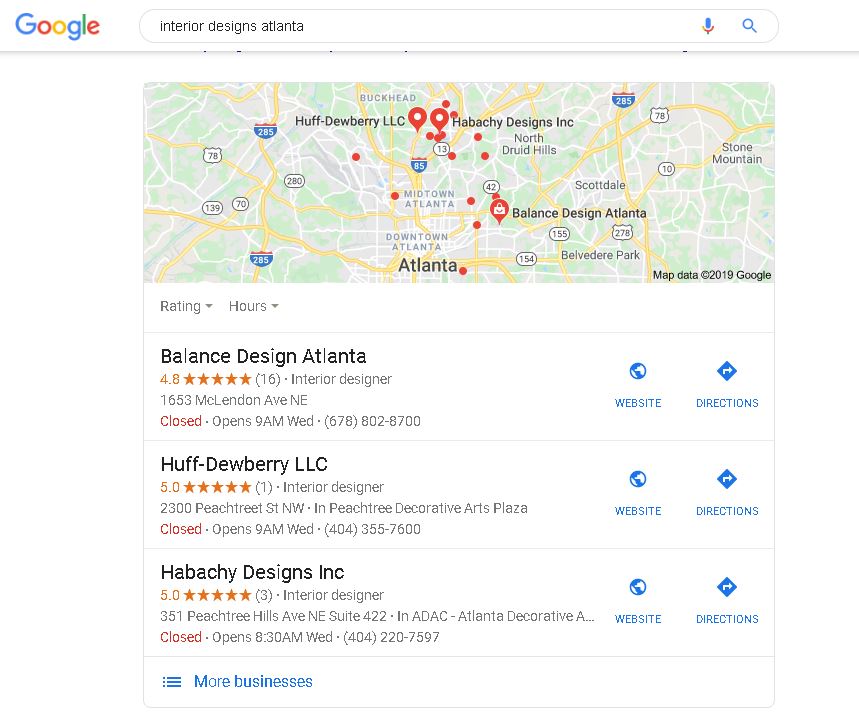This is a detailed screenshot of a Google search results page for "signs Atlanta." At the top-left corner, the familiar Google logo is prominently displayed. Centrally placed is the Google search bar with "signs Atlanta" typed into it. Adjacent to the right side of the search bar are two icons: a magnifying glass symbol on the far right, indicating the search function, and a microphone icon to its left, signifying voice search capability.

Below the search bar, a large map of inner-city Atlanta dominates the upper portion of the results page, adorned with red pin drops marking various locations. Beneath the map, on the left side, there are two drop-down boxes labeled "Rating" and "Hours" that allow users to filter their search results.

The listings of businesses start immediately below this section. The first entry is "Balanced Design Atlanta," highlighted in black text. It boasts a rating of 4.8 stars based on 16 reviews and is categorized as an interior designer. The address and hours of operation are provided below, and to the right, there are clickable icons for the business's website and directions.

The second entry lists "Huff Dewberry LLC" with a similar layout, displaying its ratings, category, address, and hours, along with icons for the website and directions to the right.

The third listing is "Hibachi Designs Inc.," which follows the same format with the website and directions icons positioned to the right.